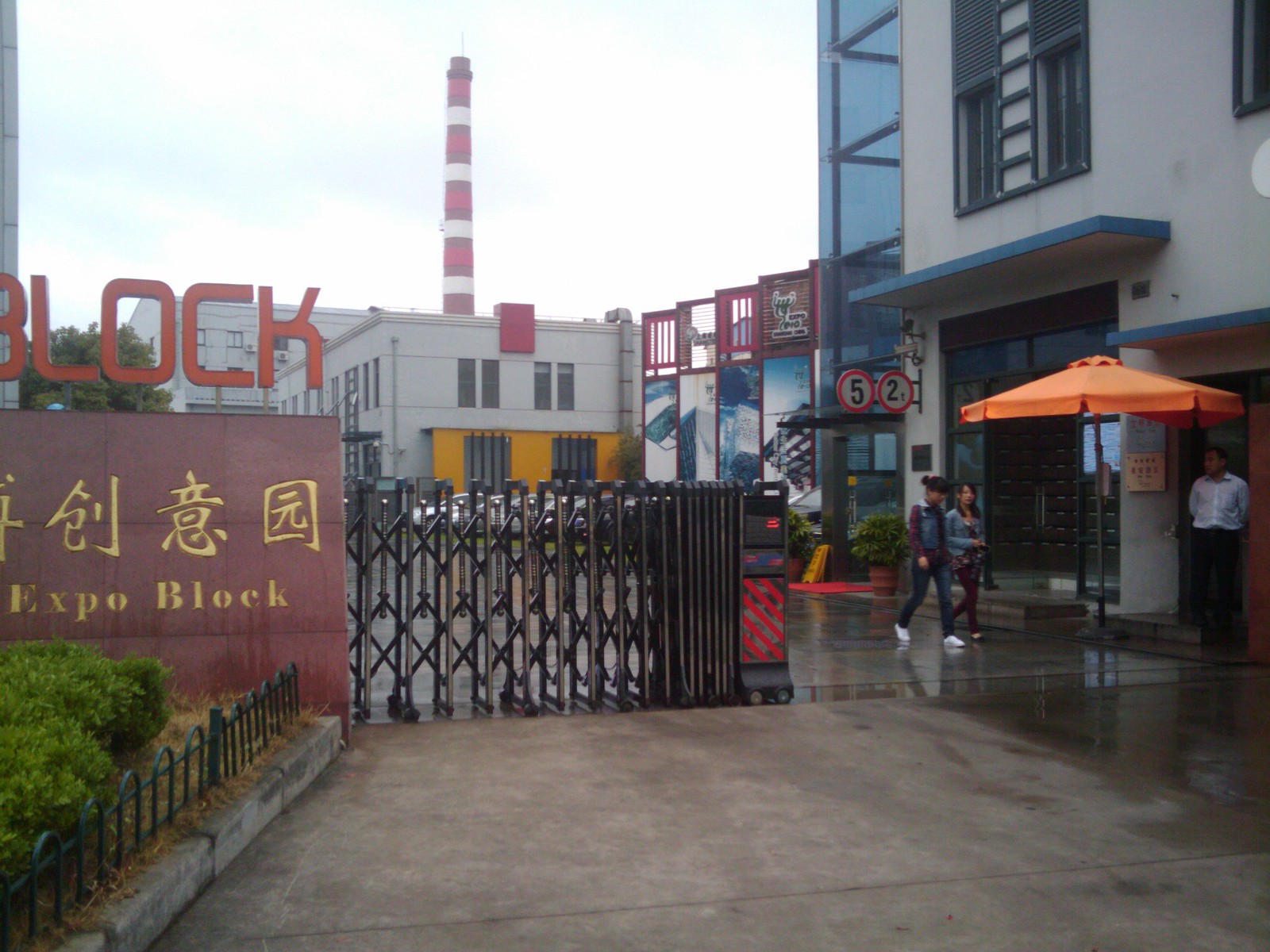The photo captures an entrance to a Chinese neighborhood on a rainy day, featuring an open electric retractable gate and an adjacent red gate barrier. On the left side of the image, there is a brown wall displaying "Expo Block" in yellow writing, with large red letters spelling "BLOCK" above it, accompanied by Chinese characters. Below this barrier, green shrubbery and a semi-circular green fence sit next to a gray curb. 

In the center, a very wet, brown road reflects the gloomy, cloudy sky. In the far background, a towering red and white-striped smokestack rises approximately 80 feet, attached to a large white building. 

To the right, there is another building with a glass façade and white exterior, identified by the number 52. An orange-topped umbrella stands in front of this building, sheltering a person underneath, while two school students walk nearby. Additional structures can be seen in the distance, including one with yellow walls and another with black and blue panels with white tops, suggesting a factory or industrial area.